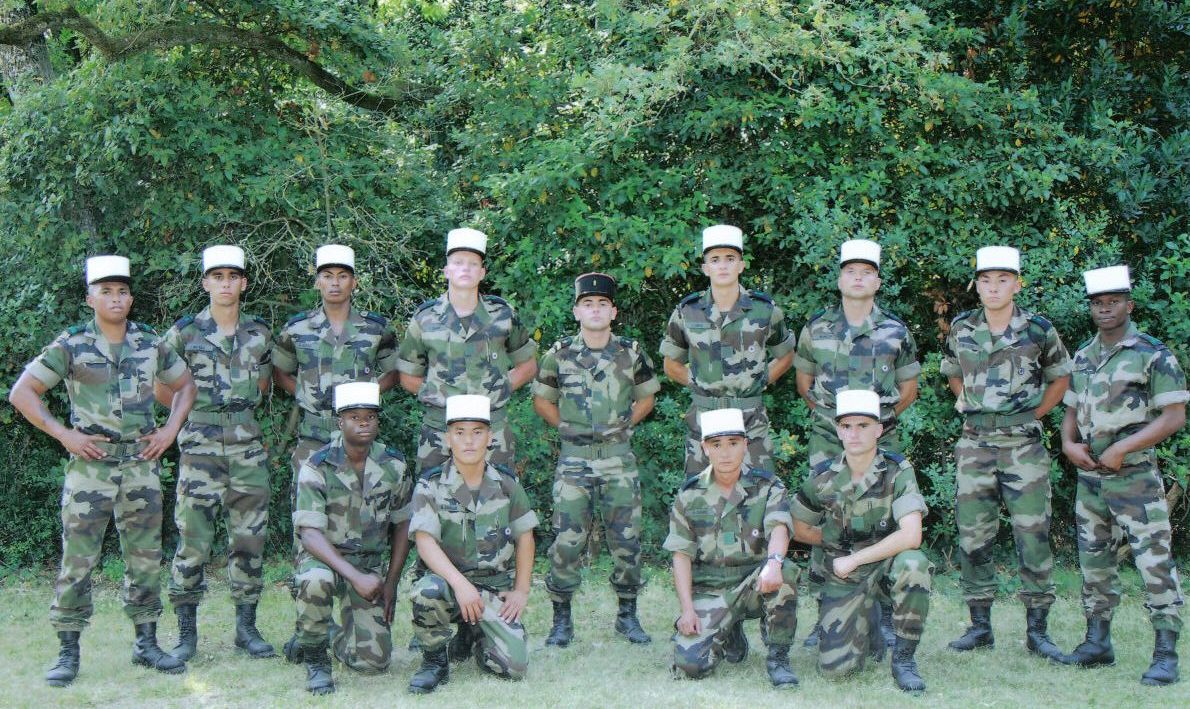This is a color photograph depicting a group of 13 young soldiers, likely in their early 20s, posing for a photo in front of a large, dense arrangement of leafy green trees. The soldiers are standing on a patchy grassy field, suggesting they might be in a cleared forest area or a grassy field. 

The soldiers are uniformly dressed in traditional green and brown Army camouflage uniforms paired with black combat boots. The group is organized into two rows: the back row consists of nine soldiers standing in a horizontal line, while the front row includes four soldiers kneeling on one knee. In the back row, the height of the soldiers ascends towards the middle, peaking with a shorter soldier at the center, and then descends symmetrically. The soldiers on the far left and far right of the back row have their hands on their hips, while the remaining ones in the back have their arms behind their backs.

All the soldiers are wearing white caps with black brims, except for the one central figure in the back row, who is distinguished by an all-black cap. The diversity among the soldiers is notable, with several appearing to be of different nationalities, including Asian, African-American, Hispanic, and Caucasian.

The photograph is wide in format and entirely free of any writing, animals, or motorized vehicles, solely focused on the group of soldiers and their natural surroundings.